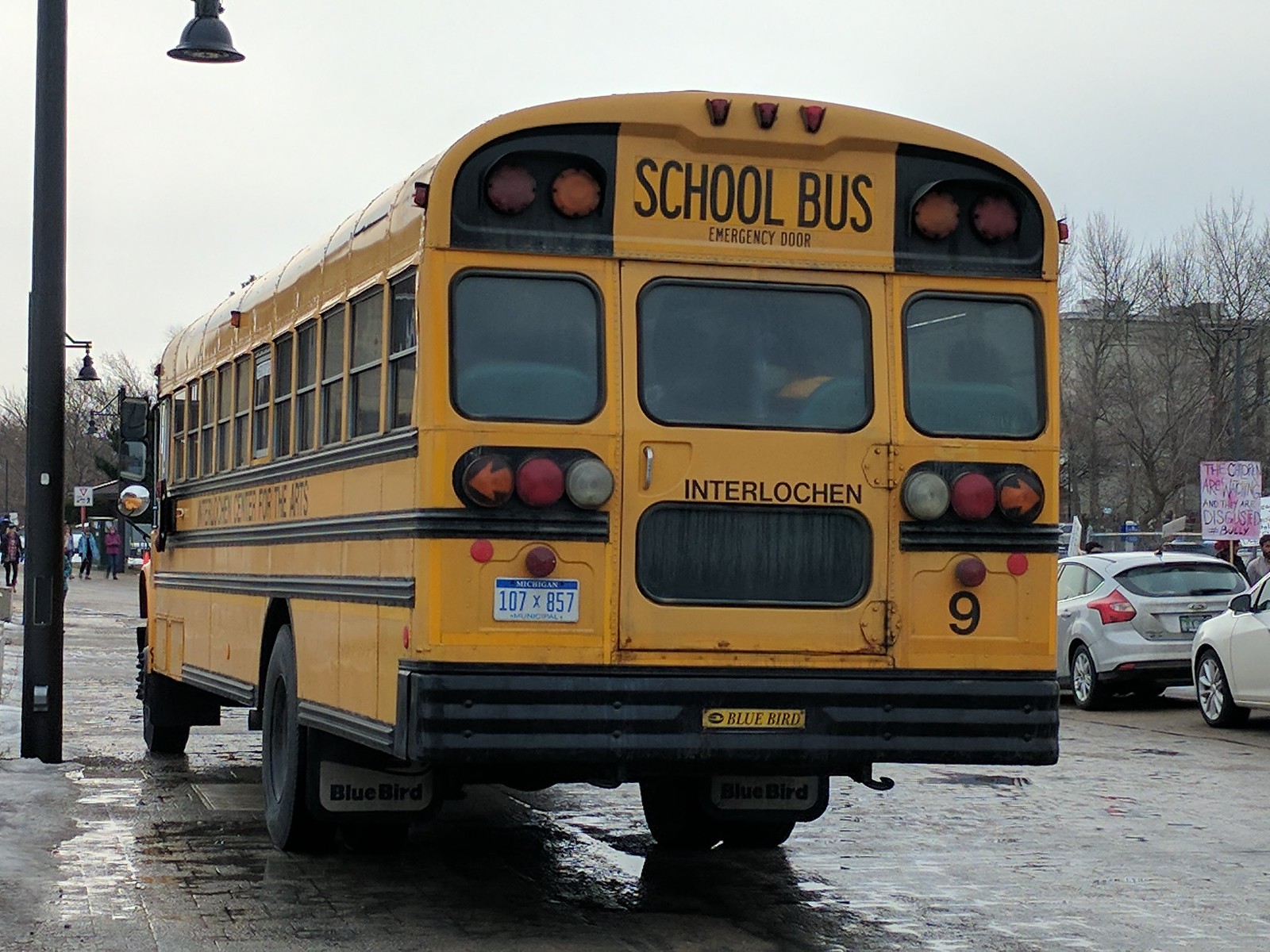The image depicts a school bus parked on a wet, cobblestone street under a light blue, cloud-covered sky. The bus is shown from the back left side, prominently displaying its yellow color and various markings, including a Michigan license plate with blue lettering against a white background and the word "Michigan" at the top. "Bluebird" is labeled on both the bumper and the tire flaps. A number nine is visible on the lower right corner of the bus. To the right of the bus, two cars are lined up one behind the other, and several leafless trees are seen in the background. The street looks wet, suggesting recent rain. Additionally, on the far right, near the background, a few people appear to be walking, some potentially carrying signs, hinting at a possible rally or protest. Overall, the scene conveys a serene yet slightly somber atmosphere, likely captured on an overcast day.